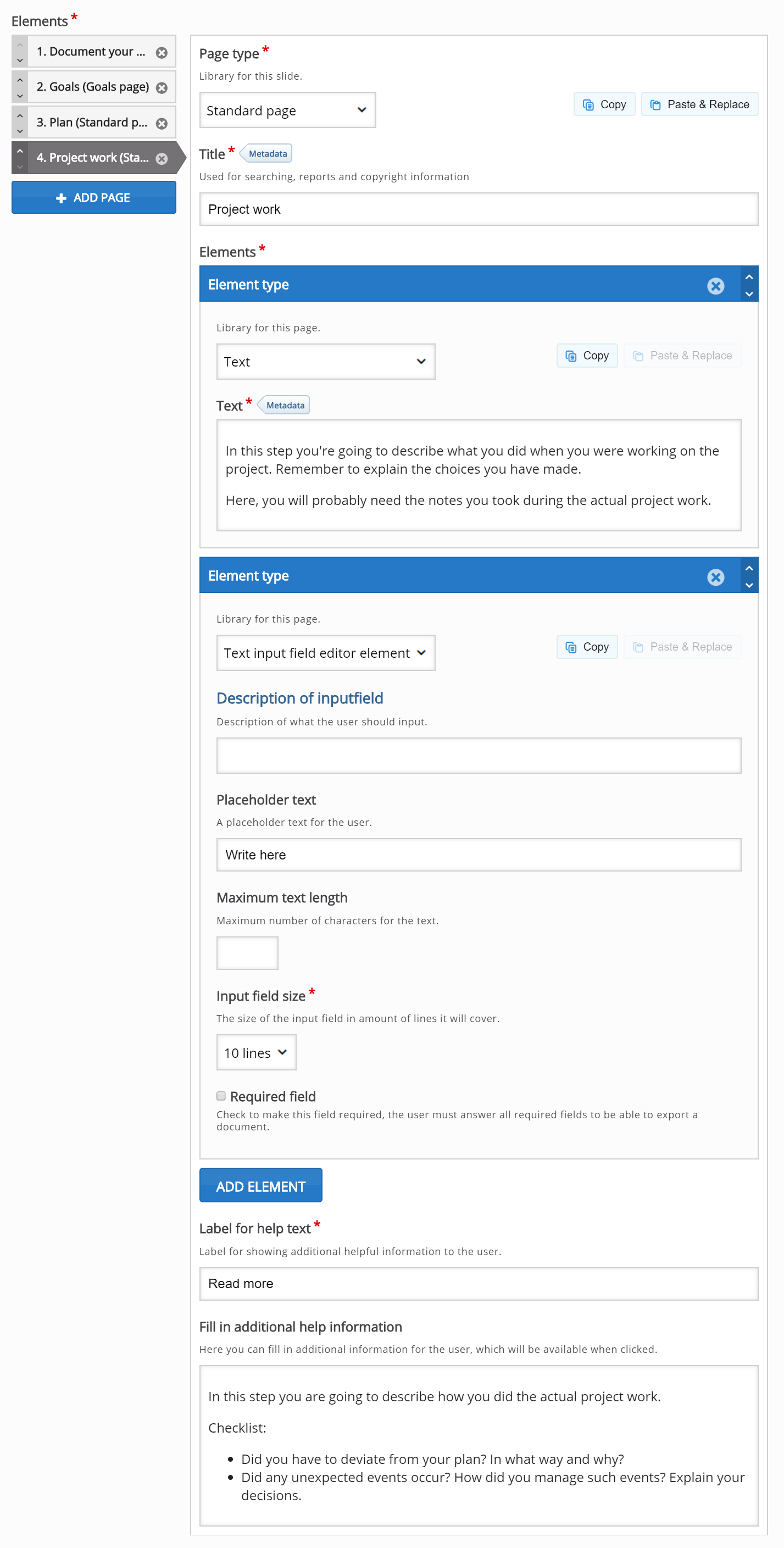A screenshot of an open settings menu is displayed on a white background. In the upper left corner, the word "Elements" is prominently written in black font, accompanied by a black asterisk. Below this, there are three smaller gray rectangles, each containing black text. The first rectangle reads "1. Document your," the second one says "2. Goals, goal page," and the third one states "3. Plan, standard." Further down, a darker gray rectangle features the white text "Project Work."

Continuing below, a blue button with white text labeled "+ Add Page" is present. Directly underneath this button is a long, vertical gray rectangle. To the right of this section, an open menu titled "Page Type" appears at the top in black font with an accompanying black asterisk. The gray text below this heading reads "Library for this site," followed by a dropdown menu displaying "Standard Page" in black font. Adjacent to the dropdown menu, two blue rectangular buttons are positioned side by side, with the first labeled "Copy" and the second "Paste and Replace," both in black text. Additionally, the menu includes the label "Title" in black font with a black asterisk, followed by the gray text "using for searching, reporting, and copyright submarines."